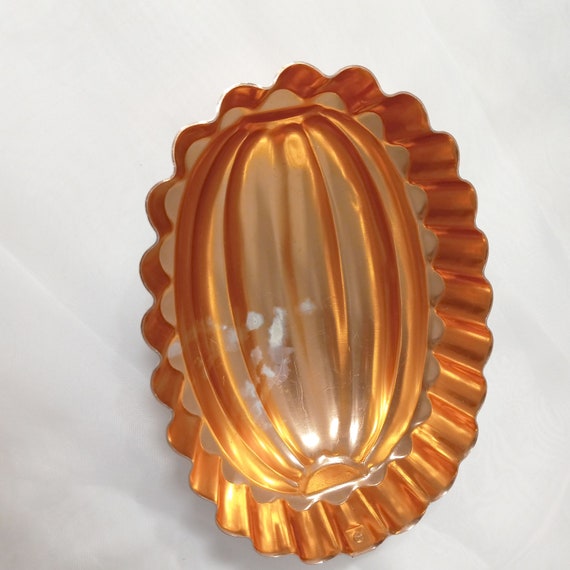The image showcases a highly reflective copper-colored mold, possibly designed for baking items such as pies or tarts. The mold features an oval shape with wavy, scalloped edges that surround its perimeter. The concave interior is adorned with a rounded, pumpkin-like or squash-shaped protrusion. The shiny, orangish surface suggests a material that could be either true copper or a metal lined with a non-stick coating to facilitate easy release of its contents. This mold is photographed from above or slightly tilted towards the camera, resting on a plain white background with some faint white residue visible on the squash-shaped section, adding to its intriguing texture.